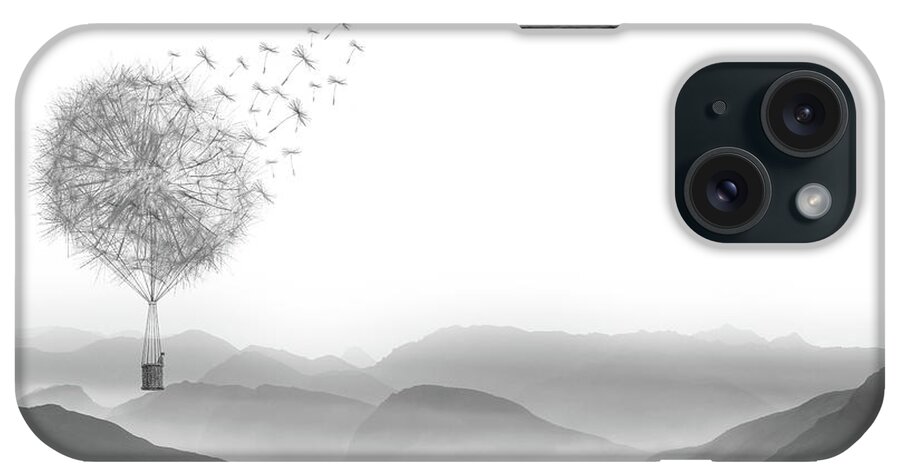The image showcases the back of an iPhone encased in a stylish, predominantly grayscale phone case. The case features a monochromatic design with shades of gray, white, and black. On the left side of the case, there's an intriguing illustration of a person sitting in a wicker basket similar to those used in hot air balloons. However, instead of a balloon, the basket is tied to a large, blown-apart dandelion, with its seeds floating away into a white, foggy sky. In the background behind the basket and dandelion, there is a depiction of a mountainous terrain consisting of various gray shades, darker at the base and lightening towards the horizon. The right side of the case reveals the phone’s dual camera lenses and flash arranged in a rounded square. The case is designed to fit the iPhone snugly, with openings for the camera, volume controls, and charging port clearly visible. The overall aesthetic is abstract and artistic, invoking a sense of whimsy and tranquility.